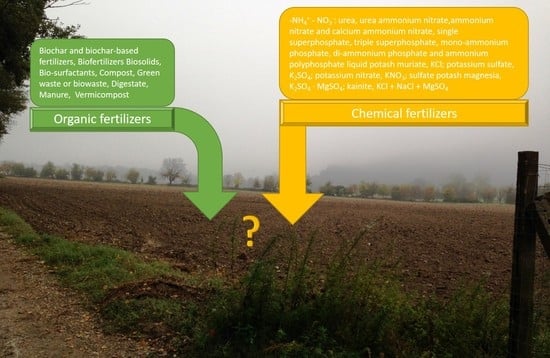The image depicts an agricultural field that has been freshly tilled and is ready for planting. Positioned in the middle of the field is a prominent gold question mark. To the right, there is a yellow sign labeled "Chemical Fertilizers" with a gold arrow pointing downward towards the soil. This sign lists various chemical fertilizers including NH4, urea, ammonium nitrate, single superphosphate, monoammonium phosphate, and potassium sulfate among others. On the left side, a green sign labeled "Organic Fertilizers" is present, also with an arrow leading down to the soil. This sign lists types of organic fertilizers used, such as biochar, biochar-based fertilizers, biofertilizers, biosolids, biosurfactants, compost, green waste, manure, and vermicompost. The field appears mostly brown with freshly turned soil, featuring sparse patches of green grass, notably more prevalent on the organic fertilizers side. This juxtaposition emphasizes the different types of fertilizers applied to each section of the field, likely for a comparative agricultural study.